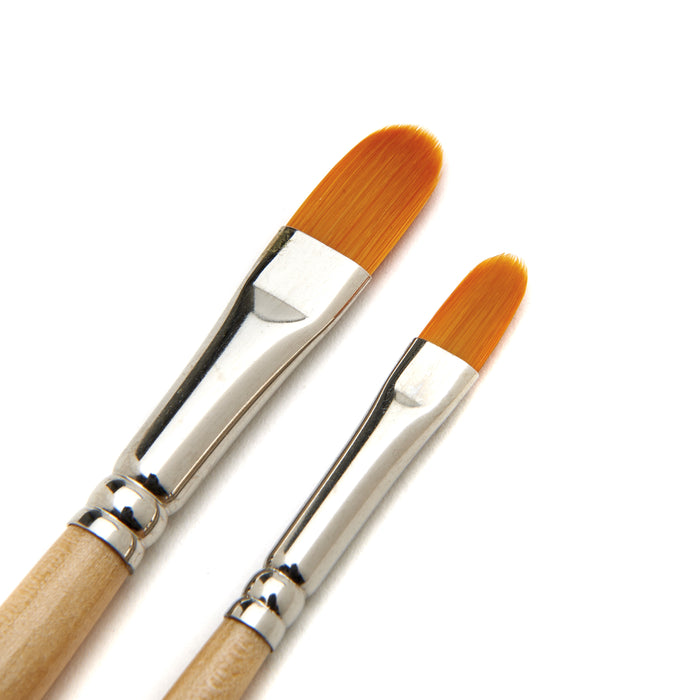The image features a close-up of two paintbrushes, potentially mistaken for makeup brushes, lying side by side diagonally against a stark white background. Both brushes are characterized by their tan wooden handles, partially visible, transitioning into shiny, silver metallic ferrules that hold the bristles in place. These metallic tops are reflective, showing hints of black and white reflections whose source is unspecified.

The bristles of the brushes are a distinct orangish-brown color and have a unique, rounded oval shape at the tip, differing from the typical flat-top design. The brush on the left is notably larger, around twice the size of the one on the right, with both sharing identical design and color features except for their size disparity. The symmetric shape of the bristles creates a rounded peak at the center, curving down gracefully on both sides. The smooth, silver ferrules reflect light intriguingly, adding a polished look to these well-crafted brushes.